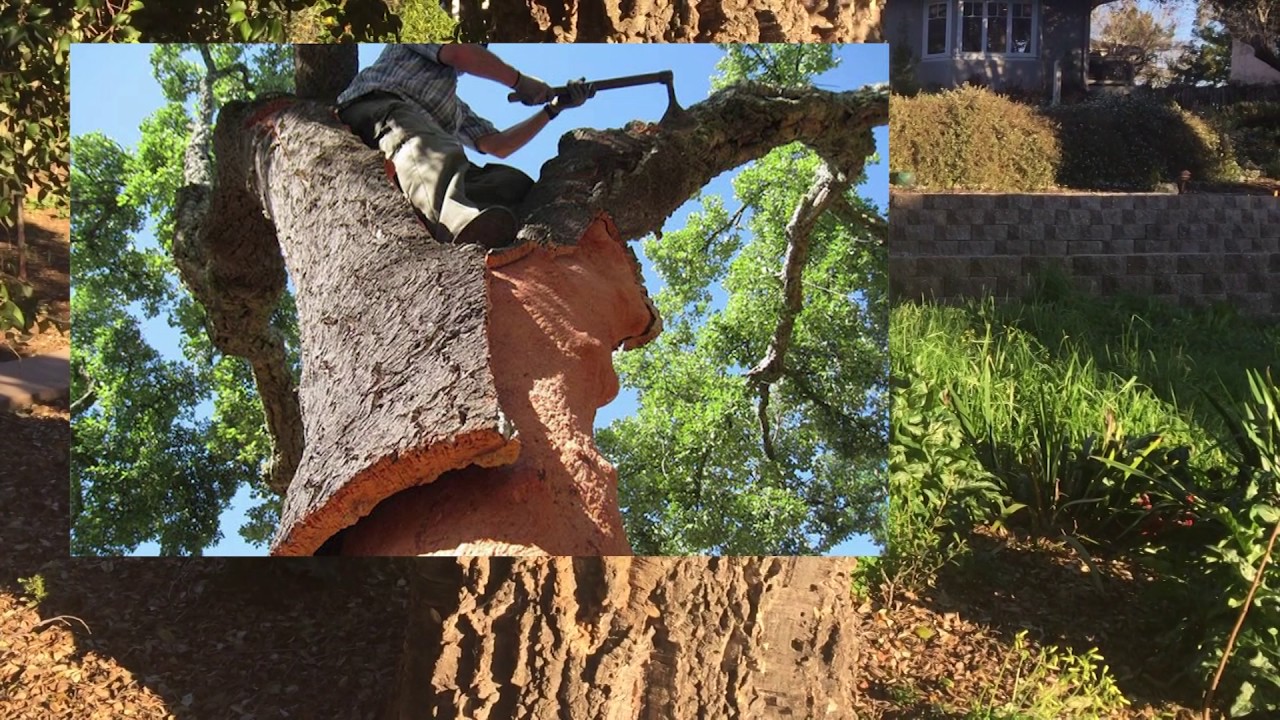This image depicts a layered photo collage with detailed elements of a backyard scene. The primary image, centrally positioned but slightly to the left, captures a man standing within the arch of a tree, taken from a low angle looking up. The man is holding a small hand axe and is actively stripping the bark from the lower part of the tree, revealing an orange clay-colored inner trunk. Surrounding this central photo, the background reveals the base of another tree, green grass, a stone flower bed, various shrubs, and a bay window of a house. Additional layered photos include glimpses of a backyard with a grey brick wall, a house facade with four windows in a row, and more greenery with deciduous trees in full leaf, all contributing to a rich, multi-faceted outdoor scene.